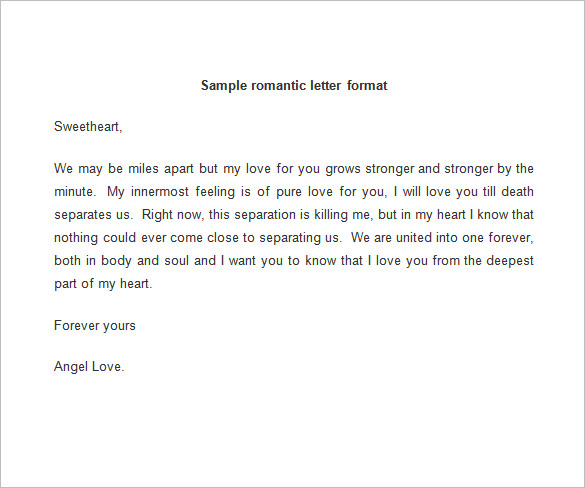The image displays a formatted sample of a romantic letter, designed to guide someone in expressing their heartfelt emotions. At the top of a black rectangular box, in black text, it reads "Sample Romantic Letter Format." The word "Sample" is capitalized. Below this, the letter begins on the left side with the salutation "Sweetheart," followed by a heartfelt message: "We may be miles apart, but my love for you grows stronger and stronger by the minute. My innermost feeling is of pure love for you. I will love you till death separates us. Right now, this separation is killing me, but in my heart I know that nothing could ever come close to separating us. We are united into one forever, both in body and soul. I want you to know that I love you from the deepest part of my heart." The letter concludes with "Forever yours," on a new line, followed by "Angel Love." The background of the image is solid white, emphasizing the letter's black text within the black box. This sample provides a clear and structured format for composing a romantic letter to a loved one.